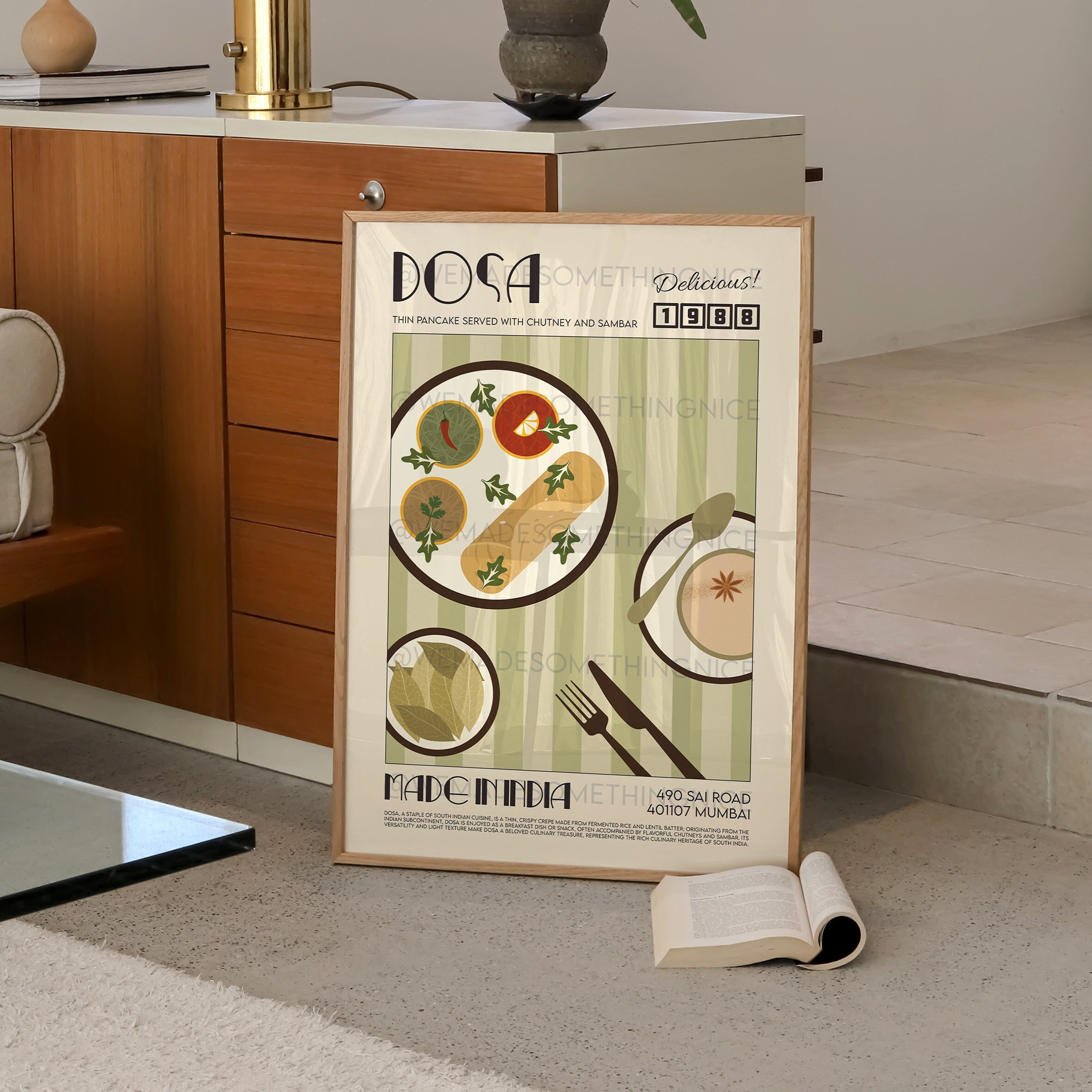This detailed image captures a cookbook cover-style poster set within a monochromatic room. The focal point is a predominantly beige poster framed in brown wood. Prominently displayed at the top are the bold black letters "DOSA" followed by the word "Delicious" and the year "1988." The caption describes "the thin pancake served with chutney and sambar," hinting at its culinary inspiration from Mumbai, India. The poster's centerpiece is a visually rich depiction of three plates of food. The top-left plate holds various food items, including bay leaves, lemons, and cups of lemon juice. Below it, another plate features just a spoon, and beside it sits a plate with a black spoon and fork. The room itself has gray tiled floors and gray walls, giving it a minimalist look. A blue desk with black front drawers and various items on top, such as a lamp, vases, and an open book, is angled from the center to the right. The photograph captures the poster leaning against this desk, further supported by another cabinet on the left. A book lies open on the floor in front of this setup. This arrangement evokes a somewhat utilitarian space dedicated to the love of cooking.